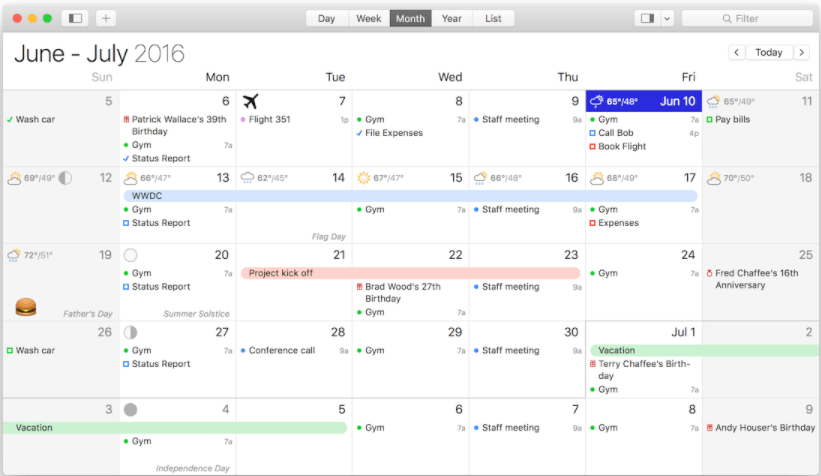The image depicts a calendar application on an Apple device, evident by the distinctive red, yellow, and green circles located in the upper left corner, characteristic of Mac OS windows.

At the top of the calendar interface, navigation options are presented: "Day" and "Week" are displayed in black text, while "Month" stands out in white text against a gray background. 

On the left-hand side, "June-July 2016" is prominently displayed, indicating the current range of dates viewed. The days of the week are abbreviated at the top, with Sunday (SUN) and Saturday (SAT) highlighted in light gray, while Monday (MON), Tuesday (TUE), Wednesday (WED), Thursday (THU), and Friday (FRI) are listed in black.

Each date is organized within individual light gray boxes. Observations begin with Sunday, the 5th of June, continuing through key dates, including the 12th, 19th, and 26th, and transitioning into July with the 3rd. The boxes for Saturdays - the 11th, 18th, 25th, 2nd, and 9th - are also noted in light gray.

Specific events are marked within the calendar:
- Hailey Houser's birthday is noted on the 9th, in black text.
- The person has a gym routine every Monday, Wednesday, and Friday.
- On June 10th, there is a reminder to "Korbach book flight."
- "Expenses" are to be handled on the 17th.
- A vacation spanning from July 1st to July 5th is clearly indicated.

The layout and notations suggest meticulous planning with color coding and detailed annotations for personal and scheduled events.